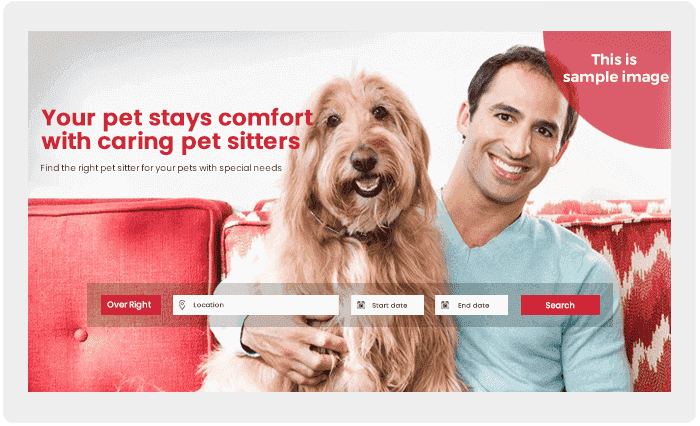This is a prototype webpage for a pet-sitting service, showcasing an advertisement for veterinarians or pet sitters. The upper right-hand corner of the webpage features a small red speech bubble icon. The sample image centers on a man seated on a red couch with a long-haired terrier. To the left of the terrier’s head is red text that reads: "Your pet stays comfortable with caring pet sitters. Find the right sitter for your pets with special needs."

The overall design appears minimalistic with a white background and several red bars. The left red bar contains options for location, start date, end date, and a search button. Some elements and text are not fully polished, indicating that this is a prototype. The page layout appears to be unfinished, with some phrases seemingly unrefined.